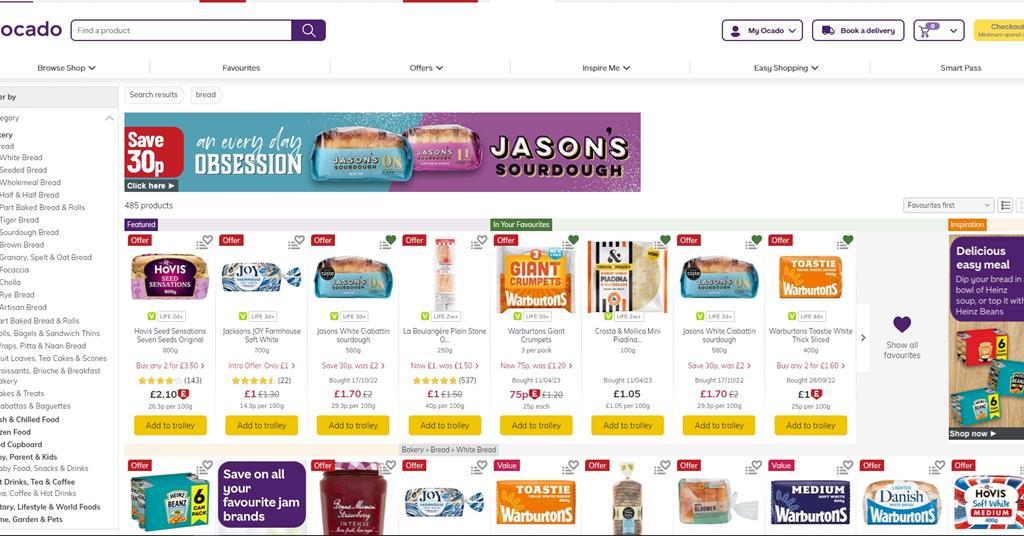The image showcases a screenshot of a grocery store website named "Ocado." The website's name is prominently displayed at the top left corner, followed by a search bar to help users find specific products. Moving to the right, users can access "My Ocado," presumably their account section, alongside options to book a delivery and view their shopping cart, which currently contains six items.

Beneath the main navigation bar are additional menu options for browsing and shopping: "Favorites," "Offers," "Inspire Me," "Easy Shopping," and "Smart Pass." Directly below these navigation options is a sidebar on the left listing various grocery categories, with "Bread" currently highlighted. The selected bread section displays various kinds of bread, each accompanied by images and details.

From left to right, the showcased breads include a loaf in a purple wrapper labeled "Seven Seed Sensation," a product called "Joy Bread," "Jason's White Sourdough Bread," an unreadable baguette, "Warburton's Giant Crumpets," a tortilla product, another "Jason's White Sourdough Bread" in a blue wrapper, and "Warburton's Toasty Thick Sliced Bread." Additional bread options are displayed below, offering a variety of sizes, prices, and packaging.